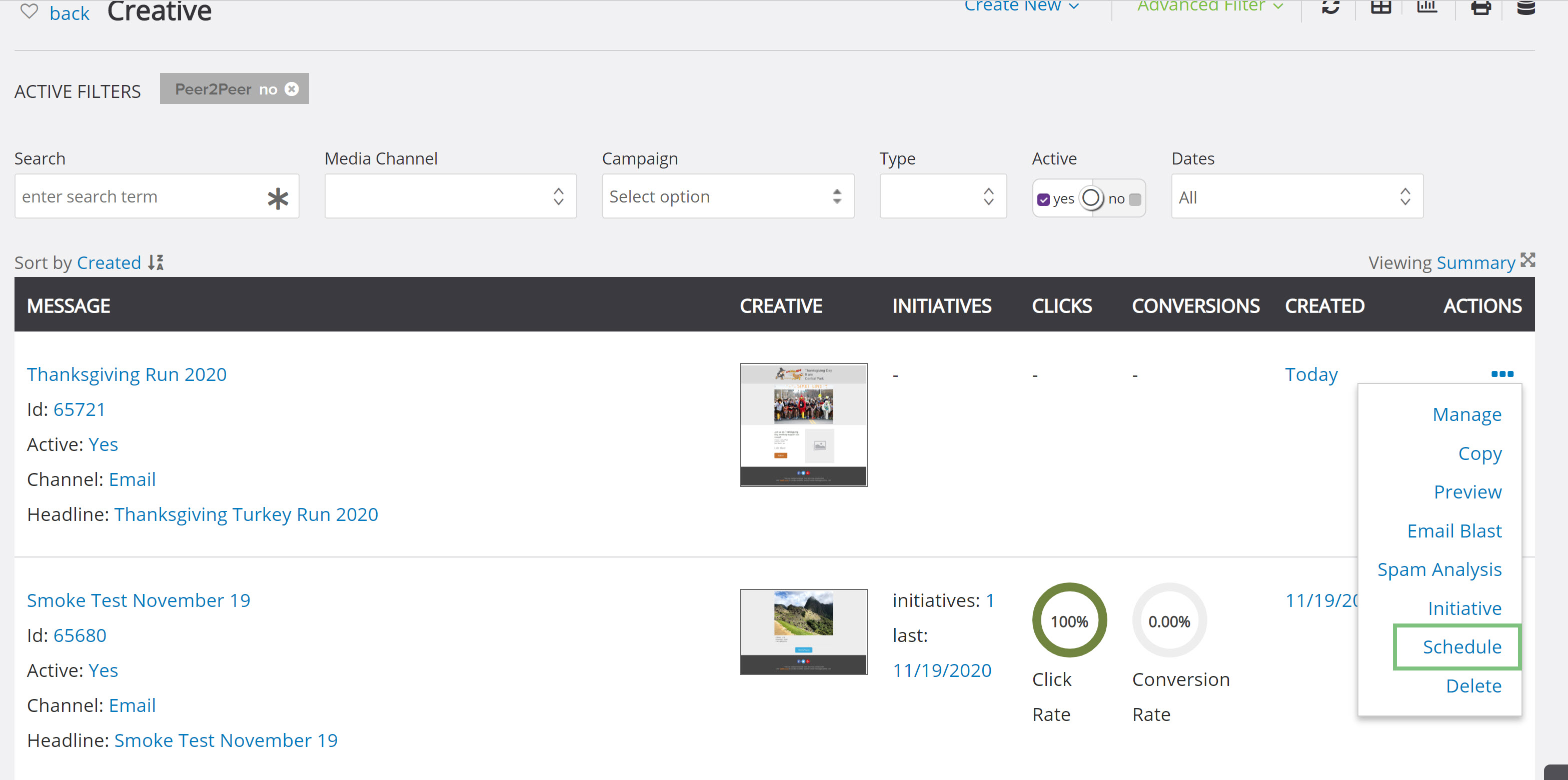The screenshot depicts a comprehensive view of a website designed for managing messages and various other functionalities. At the top of the page, the heading "Creative" is prominently displayed alongside a grayed-out button labeled "Peer-to-Peer." In the top right corner, buttons for "Create New" (in blue) and "Advanced Filter" (in green) are placed next to multiple computer icons, indicating further options or settings.

Below this section, there are several drop-down boxes for selecting different parameters: "Media Channel," "Campaign," "Type," and a date selection box. Additionally, a search bar is available for more specific queries. There is also a checkbox labeled "Active" with a binary "Yes/No" option, where "Yes" is currently selected.

Beneath these filters, a black bar labeled "Message" introduces a list of message entries. Two distinct messages are displayed:

1. The first message is titled "Thanksgiving Run 2020" and features an image, although it is indistinct and resembles another screenshot. Details for this message include:
   - ID: 65721
   - Status: Active (Yes)
   - Channel: Email
   - Headline: Thanksgiving Turkey Run 2020

2. The second message, titled "Smoke Test November 19th," includes:
   - ID: 65680
   - Status: Active (Yes)
   - Channel: Email
   - Headline: Smoke Test November 19th